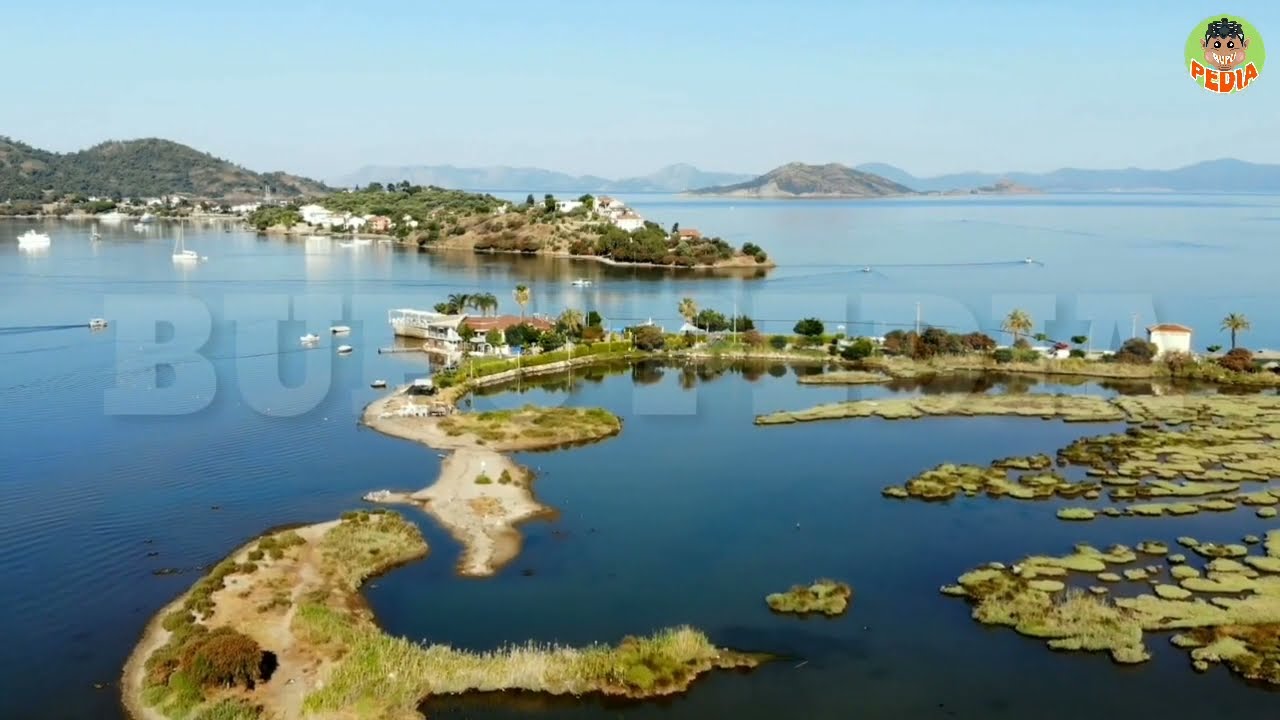The image appears to be a promotional screenshot of a tropical vacation destination, likely intended for a media brochure to entice tourists. The scene showcases an inlet leading into a bay with a docking area populated by several boats, including sailboats. Narrow islands and a developed sandbar create a patchwork landscape. One side of the inlet features a peninsula that stretches out into rolling hills, while the other side has a narrow strip of land with a road and a few buildings, possibly part of a resort. The backdrop includes mountainous islands and lush greenery with some palm trees, indicating a serene and picturesque environment. The upper right corner displays a logo with the word "Pedia" in orange letters inside a green circle, accompanied by a male cartoon character, likely the mascot. A watermark reading "buff media" spans across the image, hinting that this is a media advertisement showcasing an island retreat.